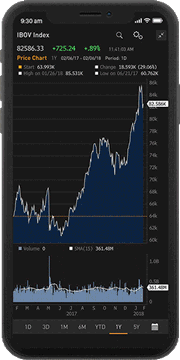The image depicts an iPhone with a black rimmed exterior featuring three buttons on the left side and one button on the right. The device's top has a noticeable line and a small dot. Displayed on the phone screen is a screenshot of a stock index, albeit slightly blurry. The status bar at the top indicates the time as 9:30 AM, with three symbols for internet connectivity and a fully charged battery.

The webpage at the top of the screen reads "IBOV Index." The upper left corner displays a value of 82,586.33, with a green highlighted number 72,524.24, showing a gain of +0.89%. The timestamp indicates 11:xx AM. Below this, "Price Chart" is highlighted in orange, followed by various metrics that are not clearly legible.

The primary chart illustrates the stock performance, starting at approximately 64% and dipping to almost 60% before sharply rising to around 76% and peaking near 84%. A smaller chart beneath this spans a longer timeframe, showing a mostly steady flow with a significant spike to the left. At the bottom, there are timeline options labeled 1D, 3D, 1M, 6M, YTD, 1Y, and 5Y, with the one-year (1Y) selection currently highlighted.